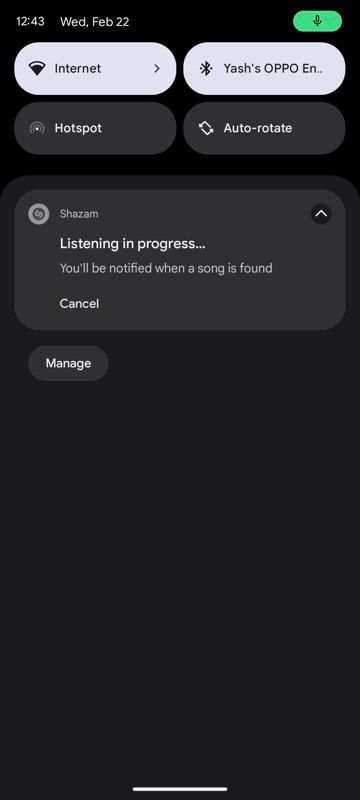This screenshot, taken from an Apple mobile device, captures a moment where the user's screen displays multiple functional elements and status indicators. 

At the bottom of the screen, the familiar horizontal white bar is visible, indicating the typical iOS navigation gesture area for exiting or switching between apps. The status bar at the top reveals the current time as 12:43 – though whether it is a.m. or p.m. is unclear – along with the date, which is Wednesday, February 22nd. The year remains unspecified.

In the top right corner, a green rectangular icon with a black microphone symbol suggests that the microphone is active. Additionally, several other status icons are displayed. The Wi-Fi indicator shows a connection strength of three out of four bars and is labeled "Internet," highlighted in a pale purplish white color. To its right is the Bluetooth icon followed by the label "YASHES's OPPOEN," indicating a connected Bluetooth device named "YASHES's OPPOEN."

Further along the top, the screenshot shows icons for additional features: an "old radio signals" icon marking the hotspot, which is currently off, and an autorotate feature that is also disabled.

Prominently, the device appears to be using Shazam, as evidenced by the display of a circular logo encompassing an 'S' lettered on its side. The screen informs that "Listening in progress" is underway, with a promise to notify the user once a song is identified. There are options to either cancel this action or manage settings related to it.

Every detail in this snapshot collectively gives a comprehensive overview of the current state and activities of the Apple mobile device.